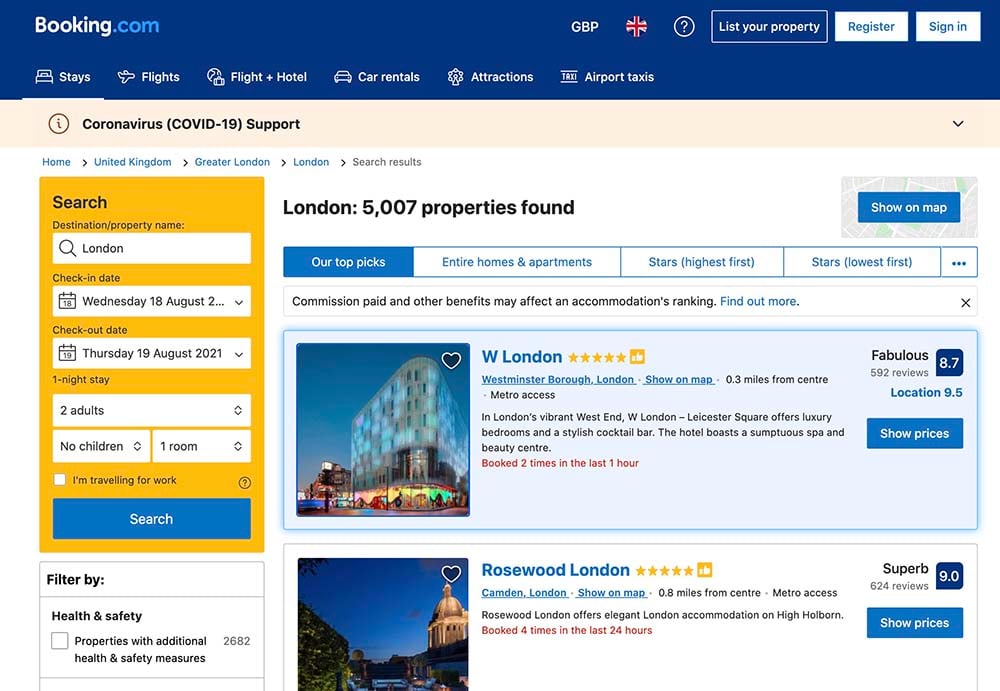The screenshot of the Booking.com website prominently features a thick blue header at the top, displaying the "Booking.com" logo on the left side. On the right side of this header, there are options for changing the currency to GBP, represented by a British flag, as well as links to "List your property," "Register," and "Sign in."

Below the header are main navigation menu options including "Stays," "Flights," "Flight + Hotel," "Car Rentals," "Attractions," and "Airport Taxis." A noticeable strip underneath provides a link to "Coronavirus (COVID-19) support."

Directly below, breadcrumb navigation shows the user's current pathway: "Home > United Kingdom > Greater London > London > Search results." 

On the left-hand side is a yellow search box prompting users to enter their destination, check-in and check-out dates, number of adults, children, and rooms, followed by a "Search" button. Beneath the search box, a filter option is available for properties with additional health and safety measures.

The main content area on the right showcases two property listings: the first being "W London" located in the Westminster Borough of London, and the second "Rosewood London," situated in Camden, London.